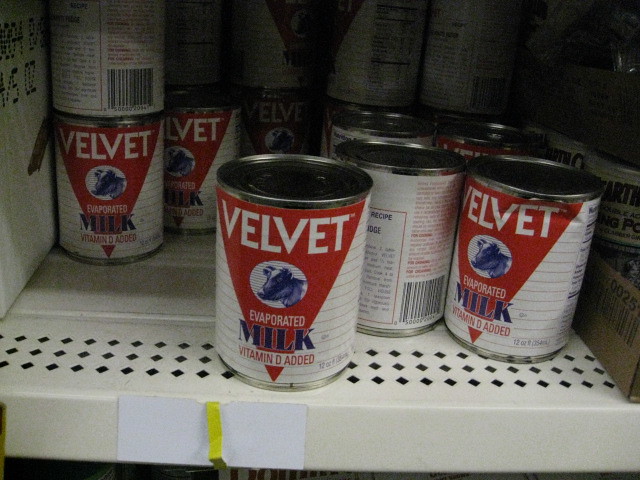A dimly lit photograph captures an interior scene of a grocery store or convenience store, focusing on a white metal shelf stocked with numerous cans. The shelf hosts about 15 identical cans of "Velvet Evaporated Milk" with added Vitamin D. The can design features a stark white background with red stripes and an upside-down red triangle. Additionally, a blue cow is prominently displayed on the label. Due to the low lighting, the upper portion of the image remains shrouded in shadows, casting a subdued atmosphere. One can on the right side of the shelf is notably dented, adding a touch of imperfection to the otherwise orderly display.